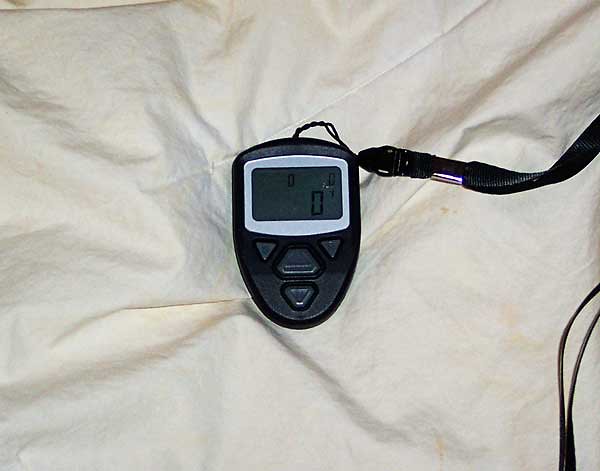A detailed photograph of a black plastic stopwatch resting on a yellowed, light-colored fabric. The stopwatch has a unique shape, starting as a slight rectangle at the top and tapering into an oval at the bottom. An LED screen, framed in silver, prominently displays three zeros ("000"). Four buttons adorn the device: two black triangles pointing downwards on the outer edges and two rounded triangles in the center, with one pointing up and the other pointing down. A black woven lanyard is attached to the stopwatch, adding to its functionality and ease of use.